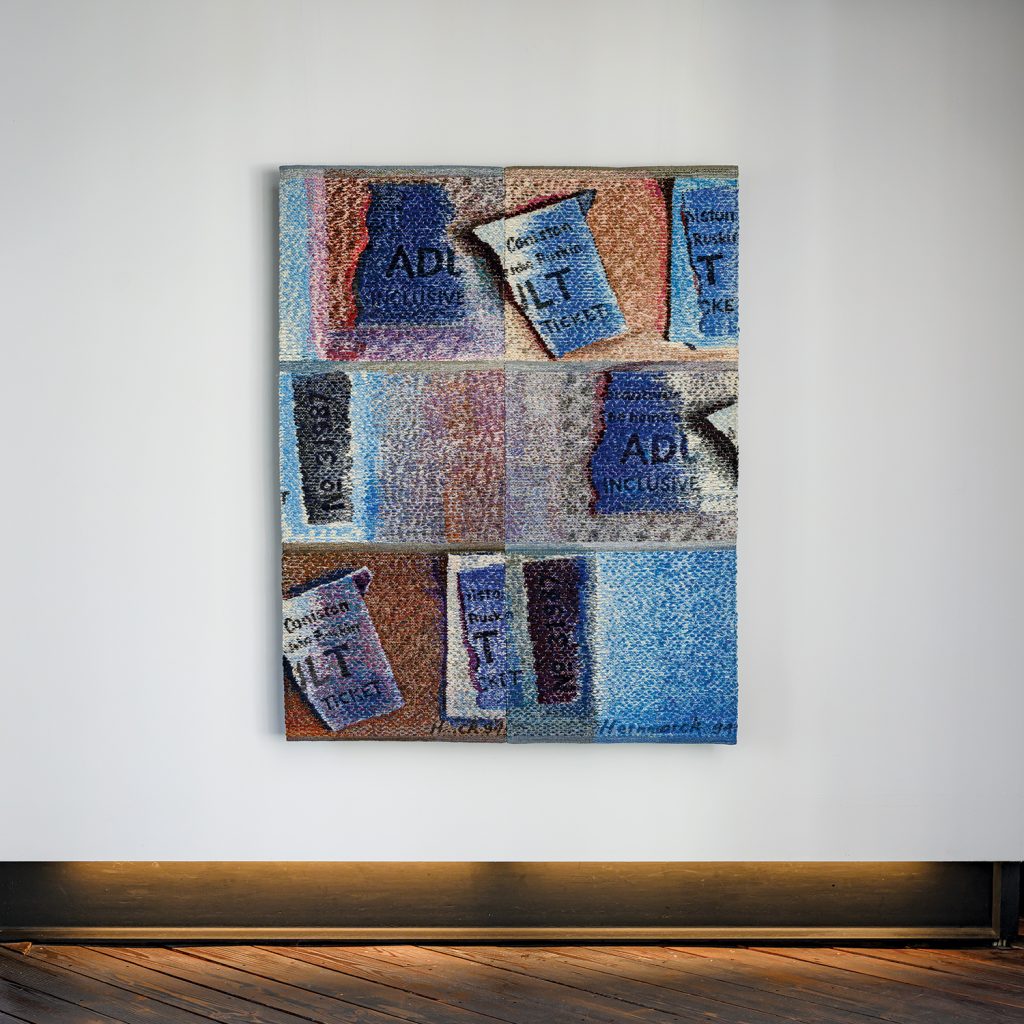This image features a piece of artwork prominently displayed on a light gray wall, accented with a dark brown border at the bottom. The wooden plank flooring beneath the wall is laid diagonally and has a polished brown finish. The artwork, a rectangular painting oriented in portrait mode, is composed of a patchwork of colors and patterns reminiscent of worn denim. Dominated by hues of dark blue, light blue, brown, black, gray, and white, the painting includes various hazy and blurred patterns. Scattered throughout the design are elements resembling torn tickets, upon which words like "31987" and "Coniston" are visibly inscribed. These ticket fragments are arranged in a way that suggests a larger, deconstructed form. At the very top, a prominent torn ticket-like shape stands out in different shades of blue. The intricate design of the painting creates an illusion of it being woven, with its six distinct panels forming a two-by-three grid, each panel showcasing part of the fragmented tickets. Finally, at the bottom of the painting, the artist’s watermark reads "Anna Rock, 1994."